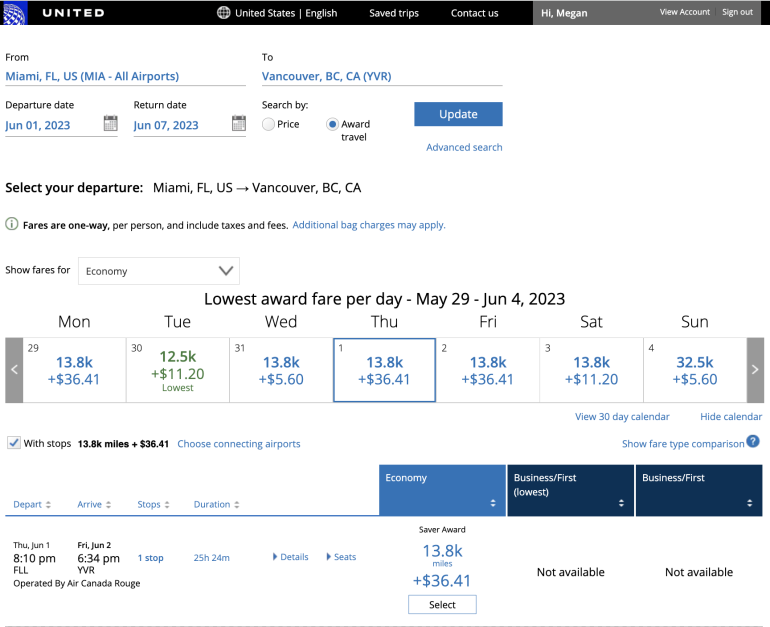The image showcases a United Airlines flight booking webpage. At the top right corner, the user's name "Megan" is displayed, with options to view the account or sign out. The page encourages safe trips and offers a 'Contact Us' link for assistance. The booking details indicate a trip from Miami, Florida to Vancouver, with a departure date set for June 1, 2023, and a return date of June 7, 2023. Users are prompted to search for travel options and select their preferred departure. Available travel classes include Economy and Business First, with a saver award option highlighted.